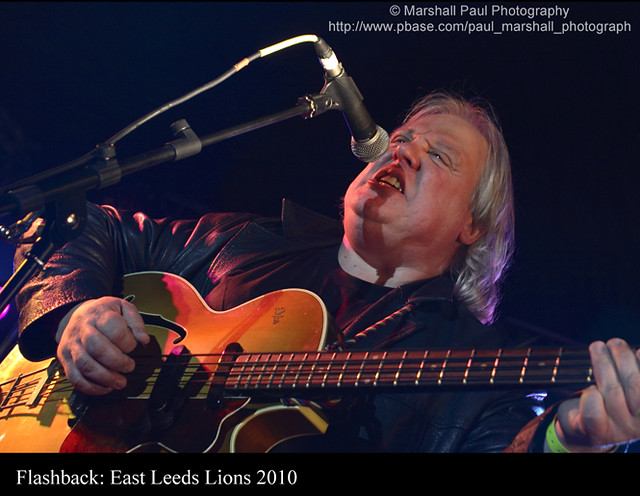In this photograph, an older white man, likely in his 60s or 70s, with shoulder-length gray hair, is captured in the midst of a performance. He is wearing a black leather jacket and playing a wooden-finished acoustic guitar. The man is leaning back, singing into a silver and black microphone positioned directly in front of his mouth. The background is stark black, making the details pop. In the upper right-hand corner, the photo attributes read "Marshall Paul Photography" with a website listed as "www.pbase.com/PaulMarshallPhotography." The lower left-hand corner of the image bears the subtitle "Flashback East Leeds Lions 2010," suggesting the photo was taken during a performance by this band in 2010.